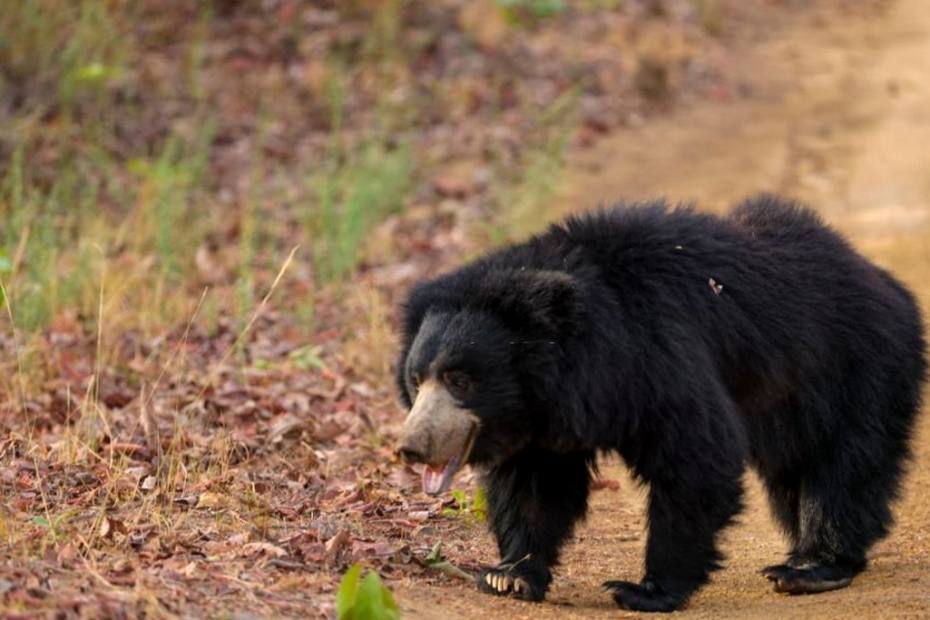In this captivating wildlife photograph, a black bear, seemingly a cub with a long, dense fur coat and a tan snout, roams towards the right side of the frame on a dirt path dotted with brown fallen leaves. Its mouth is open, possibly revealing signs of thirst or hunger. The bear, appearing slightly skinny and perhaps in search of food or its parents, exhibits a curious demeanor with wide eyes and a protruding tongue. The surrounding environment, primarily consisting of earthy tones with patches of green grass amidst the dominant brown foliage, enhances the natural, forest-like setting. The bear's paws, with visible little toes, add an intricate detail to this rich portrayal of wildlife, emphasizing the untamed essence of the creature in its habitat.